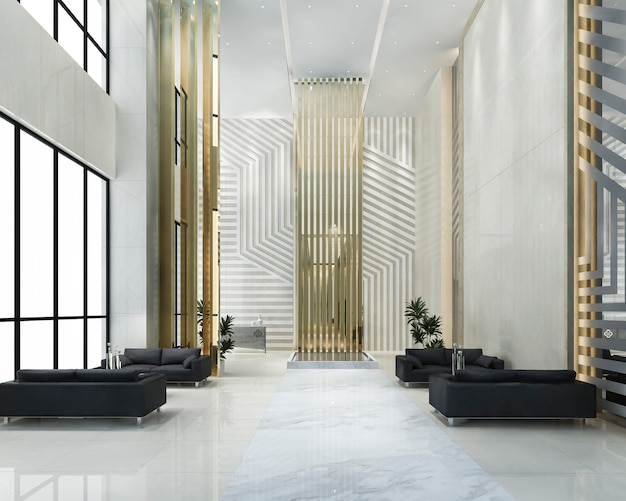The photograph captures an expansive lobby of what appears to be a commercial building, possibly an office or a hotel. The ceiling is notably high and painted white, adding to the room's grandiosity and modern aesthetic. The color palette is a sophisticated mix of white, black, gold, and silver, and the décor hints at an 80s revival of Art Deco with sleek, circuit-like lines. Central in the background are towering gold bars that extend from floor to ceiling, creating a striking focal point. On either side of the lobby, four black couches are symmetrically placed—two on each side—with two facing large, opaque floor-to-ceiling windows adorned with black vertical lines. On the left side, gold pillars add a touch of luxury, while translucent windows with intricate etchings float to the right, suggesting an entryway to another room. The floor is polished marble, enhancing the room's elegant and stark atmosphere. Additionally, a couple of potted palms bring a hint of greenery to the sleek, metallic surroundings.